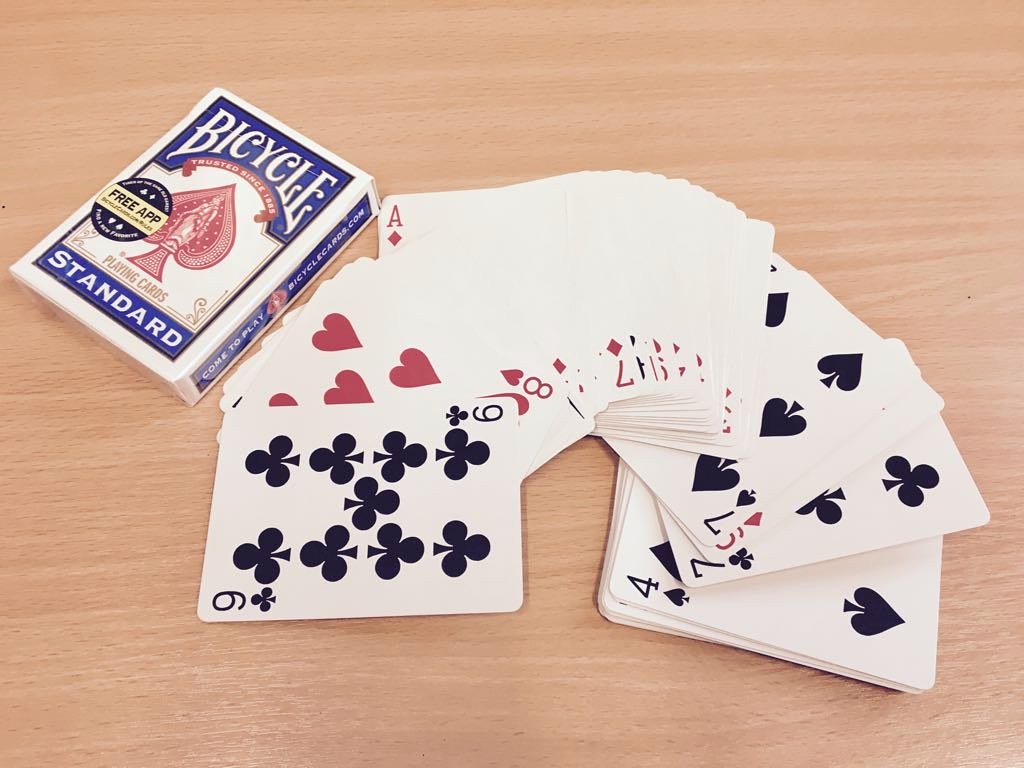The photograph showcases a spread of playing cards arranged on a wooden table. In the top left corner, the box from which the cards were taken is partially visible. The box is marked with the "Bicycle" brand, known for its slightly ornate, white font against a blue background. The box indicates the brand's long-standing reputation with a red banner that reads "Trusted Since 18--" (the exact year is partially obscured). Beneath the banner, a red spade symbol is prominently displayed. In gold letters below the spade, it states "Playing Cards," and further down, in white letters on a blue background, it reads "Standard." Additionally, there is a circular logo on the box, featuring a gold banner that advertises a "Free App."

The playing cards are fanned out across the table. The nine of clubs, characterized by its black suit, is prominently placed at the top. Behind it, the eight of hearts is partially visible. The ace of diamonds, identifiable by its red suit, peeks out from the bottom of the pile. Other cards in the spread include the seven of clubs, which becomes visible towards the opposite end. Several other card pieces and numbers are partially obscured within the fanned arrangement, adding to the intricate detailing of the scene.